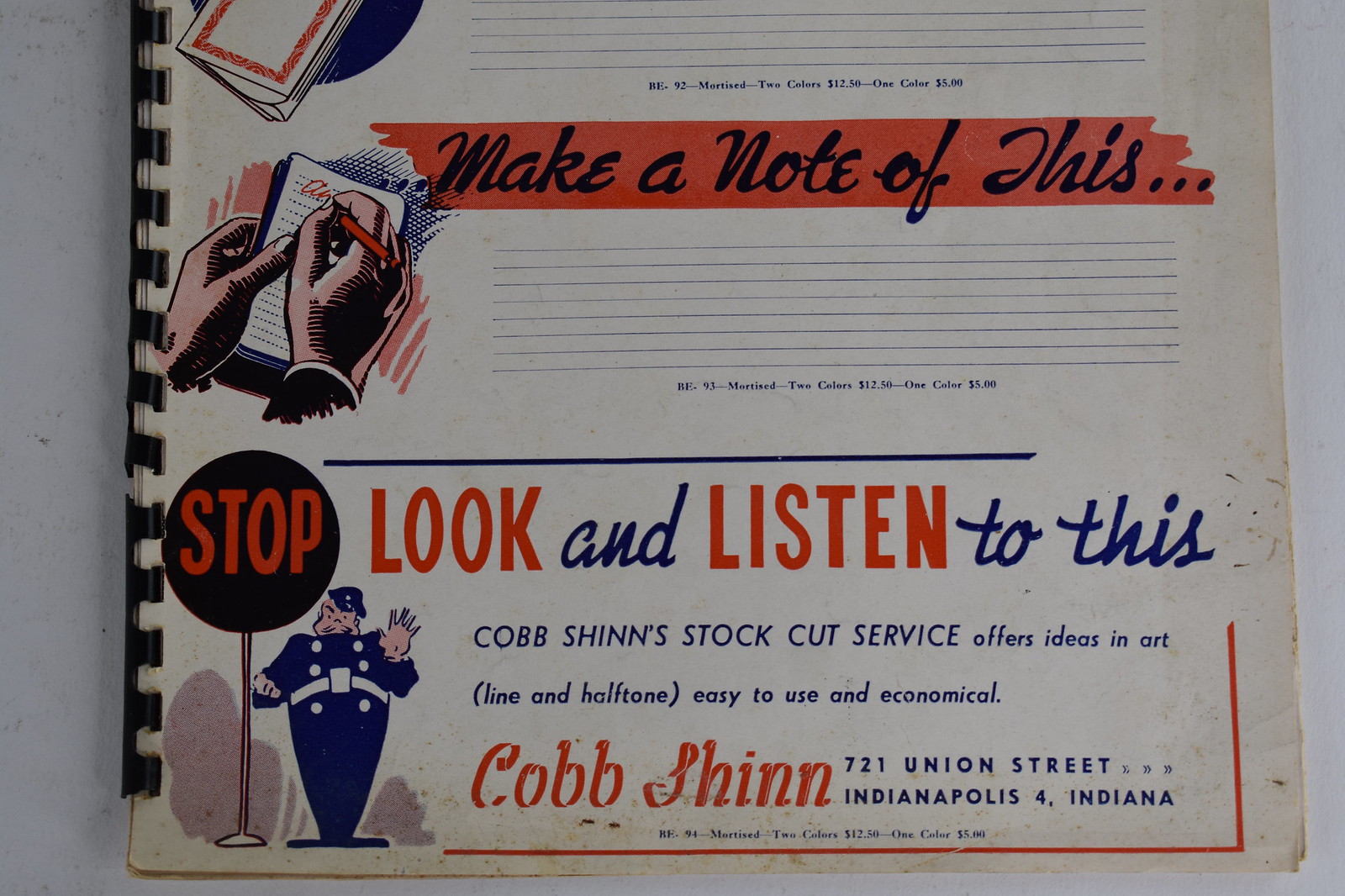The photograph depicts a hardcover notebook, bound with a black plastic strip rather than a traditional spiral. The cover is densely illustrated with various elements. On the top, a red banner reads "Make a note of this..." in black font. Below are blue lines intended for writing, and to the left, a cartoon hand is depicted writing in a notebook with a red pen. Further down, another illustration shows a stout police officer in a vintage blue uniform, complete with white buttons and a large white belt, holding a stop sign. The sign is unusual as it's circular with "STOP" in red letters. Next to the officer, italicized text reads "Look and listen to this" with "look" and "listen" in red, and "to this" in blue. Beneath this, blue text proclaims "Cobb Shinn's Stock Cut Service offers ideas in art, line, and halftone, easy to use and economical." Finally, in a cursive red font, "Cobb Shinn" is repeated with the street address "721 Union Street, Indianapolis, Indiana" written below in blue.